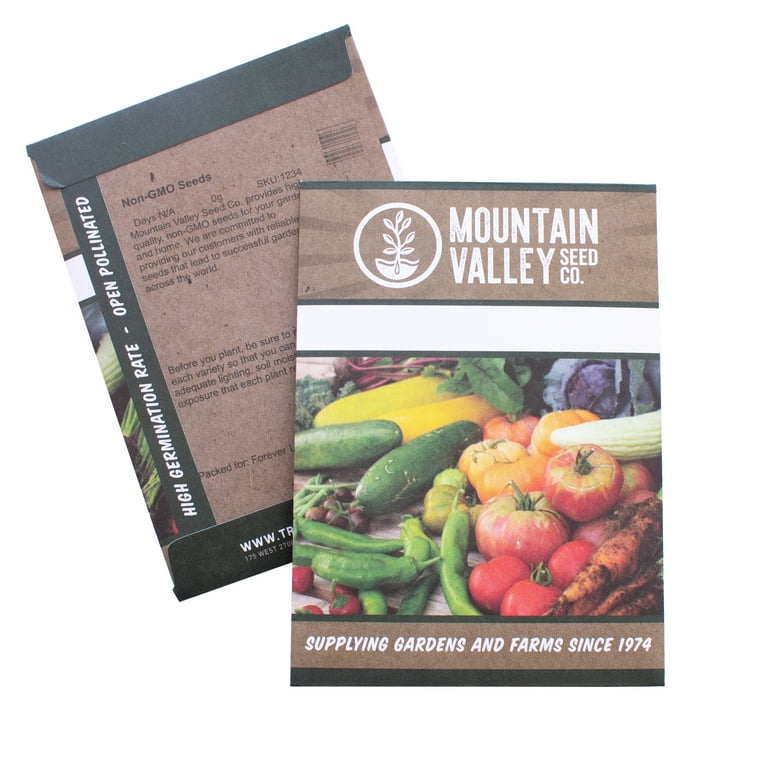The image showcases both the front and back sides of a seed packet from Mountain Valley Seed Company. On the front, it prominently displays the company's logo and slogan, "Supplying Gardens and Farms since 1974." The design features a beige and purplish border at the top with white lettering and a white bar beneath. Below this, a vibrant photograph captures a variety of fresh vegetables, including squash, zucchini, cucumbers, peppers (both green and orange), tomatoes, carrots, purple cabbage, corn, and possibly beets or turnips. The back of the packet, seen behind the front, has a brown background with black text and accents of green and white. It highlights key details like a high germination rate, open-pollinated, and non-GMO seeds. Additional elements on the back include planting instructions, a partially visible web address starting with "www.tr," and a barcode with the SKU number 1234.